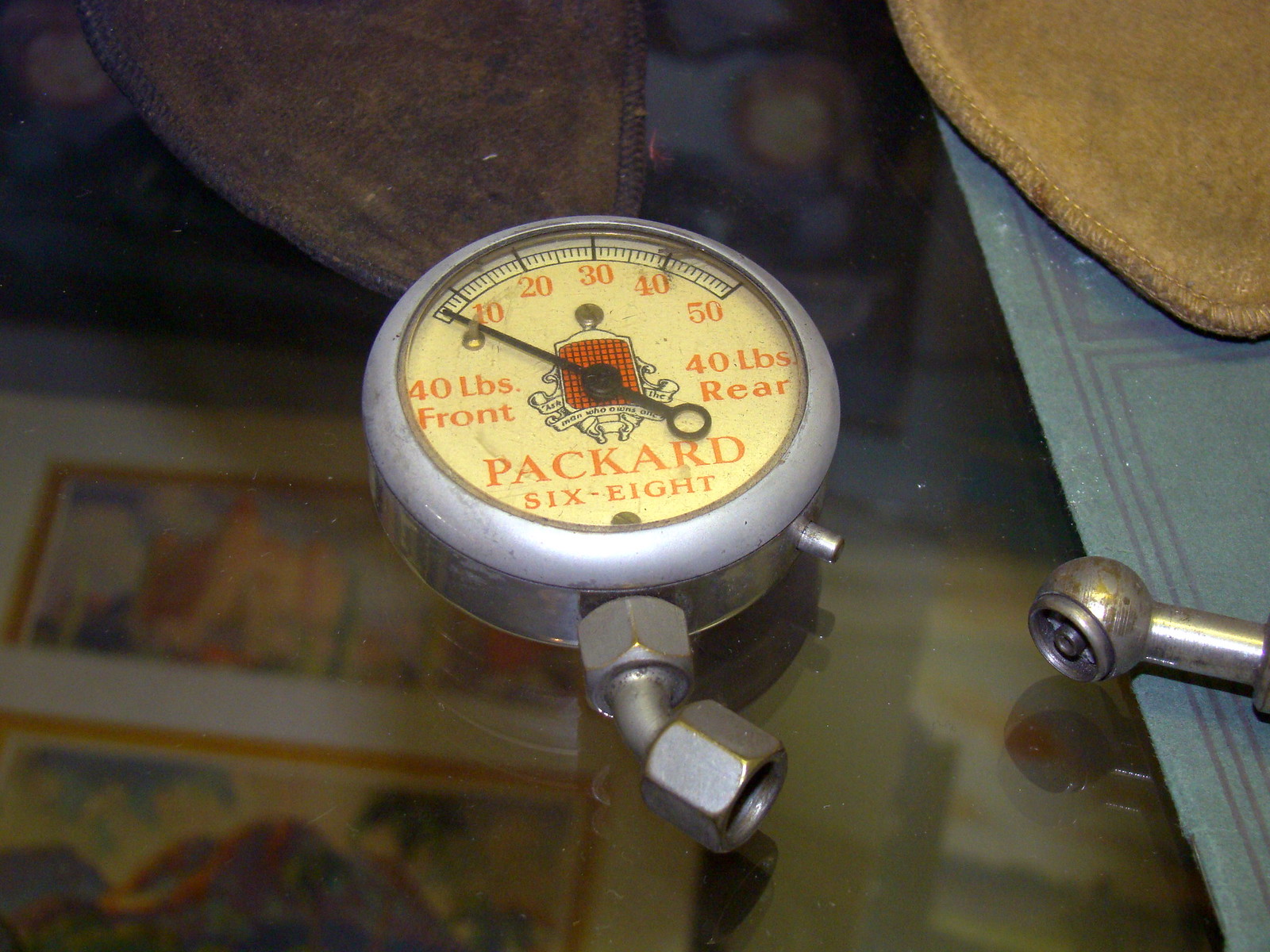A vibrant, detailed color photograph showcasing a chrome-colored pressure gauge elegantly resting on a glass surface. The gauge features a prominent yellow face, marked with a black arrow and pressure readings ranging from 0 to 50. On the left side in bold red letters, "40 pounds front" is displayed, while on the right, it reads "40 pounds rear." At the bottom of the gauge, the label "Packard 6.8" is clearly visible. The right side of the image includes the tip of a tire gauge, typically used for checking tire pressure, hinting at the gauge's utility. In the upper right-hand corner, part of a brown leather object, adorned with visible stitching, peeks into the frame. Through the glass surface, a series of color photographs add depth and background interest to the composition.